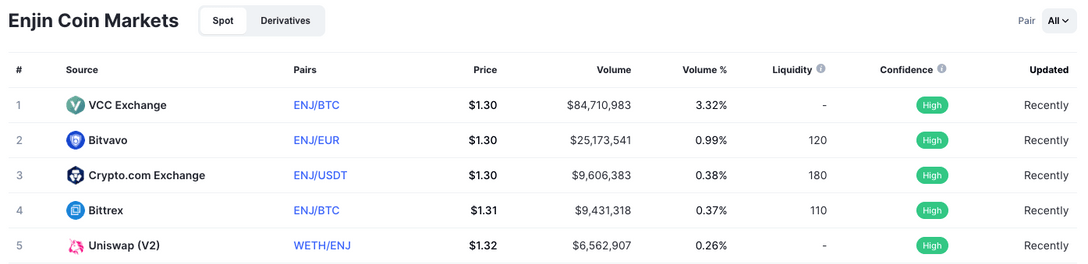This horizontal screenshot, set against a solid white background with subtle gray accents, showcases a detailed view of a cryptocurrency platform. Dominating the upper left corner is the text "Engine Coin Markets" in large, bold black font. Adjacent to this, on the right, is a gray box featuring a smaller white box inside, labeled "Spot and Derivatives" suggesting selectable options.

Below the "Engine Coin Markets" heading is a vertical column starting with the pound sign (#). To the right of this column is the header "Source." Each row beneath lists various cryptocurrency exchanges from 1 to 5. The first row displays "VCC Exchange" marked with a small green circle containing a white "V" to its left. The subsequent rows list “Bitbavo” as number 2, “Crypto.com Exchange” as number 3, “Bittrex” as number 4, and “Uniswap” as number 5.

Towards the upper right side of the screenshot, a gray button with a pull-down arrow labeled "All" suggests filter or sorting options.